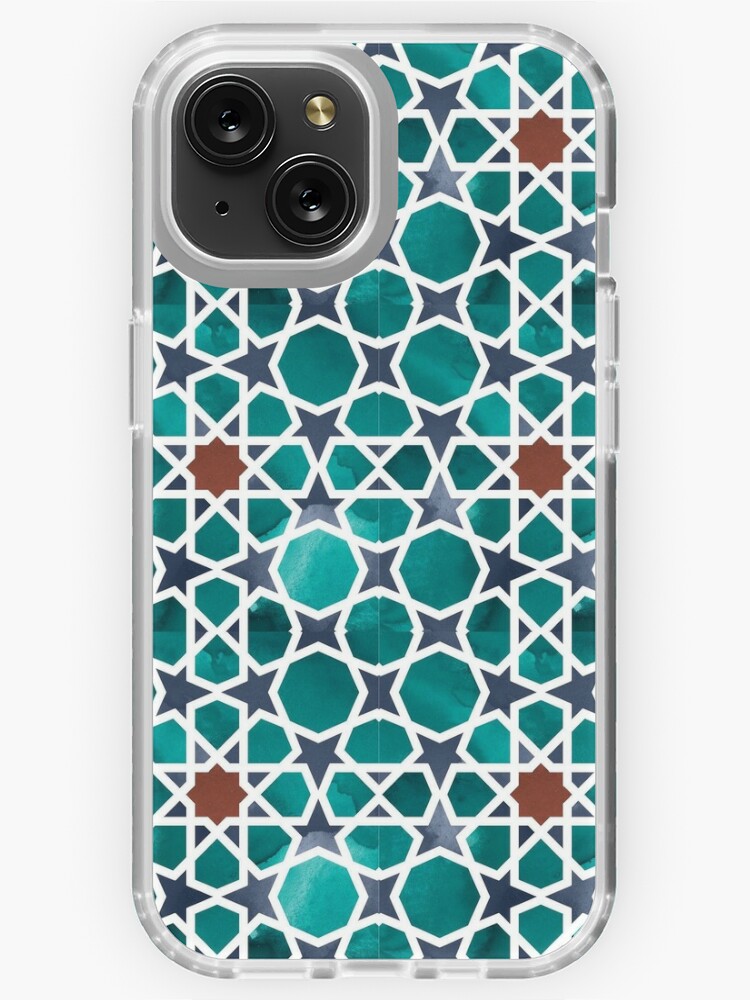The image features an iPhone placed on a white surface, showcasing the back of the device encased in a geometric-patterned cell phone case. The phone case is adorned with a variety of shapes, including stars, hexagons, pentagons, and other abstract figures, outlined in white. The colorful pattern includes green, gray, and red hues, with green being more predominant in the larger shapes, and gray and red in the smaller star-like figures. The iPhone itself has a silver-colored frame, emphasizing its camera setup. The camera area, located in the upper left corner, is encapsulated in a silver border for protection. The camera includes two lenses, one in the upper left and one in the lower right, complemented by a small gold button on the upper right and a black button on the lower left, all set against a black background. The phone case also features white columns running vertically along the sides and horizontally across the middle, bottom, and top of the phone. The detailed pattern and silver accents add a unique, visually appealing aesthetic to the device.